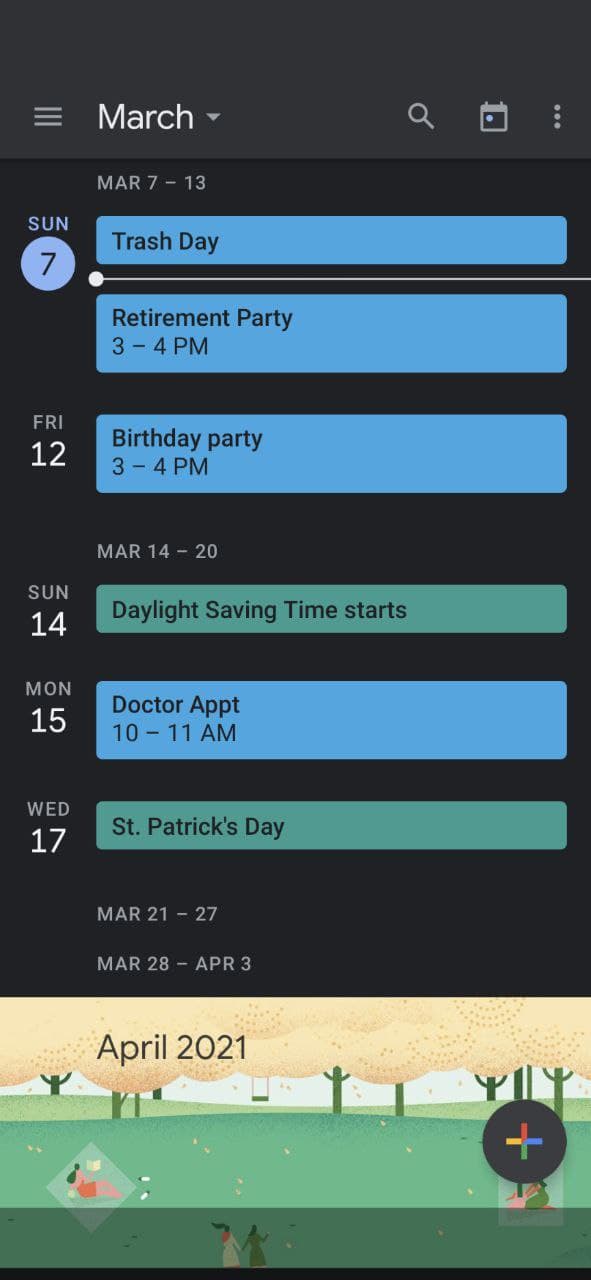The image is a phone screenshot showcasing a calendar application. At the top of the screen, three horizontal lines, known as the hamburger icon, are visible. To the right of these icons is the month "March" with a small drop-down arrow next to it, indicating the possibility to change the month view. Further to the right, near the middle, there is a magnifying glass icon followed by a calendar icon, and then a three-dot menu icon. This top bar area is shaded in a light gray color.

Below this section, there is a black background area displaying the week of March 7th through 13th. The 7th is circled in a light purple color, indicating the current date. Adjacent to the date, there is a rectangular light blue box labeled "Trash Day." A horizontal line separates this entry from another event, "Retirement Party," scheduled from 3 to 4 p.m., also in a light blue rectangle.

Towards the bottom left, for Friday, March 12th, another event is listed: "Birthday Party" from 3 to 4 p.m., highlighted in a light blue rectangle. Underneath this event is the week of March 14th through 20th. This section includes an entry in a light green rectangle that reads "Daylight Savings Time Starts," specifically on Sunday, March 14th. Additional days listed under this week include Monday the 15th and Wednesday the 17th.

At the very bottom, the image notes "April 2021" along with a cartoonish drawing of a forest, adding a whimsical touch to the otherwise structured calendar view.